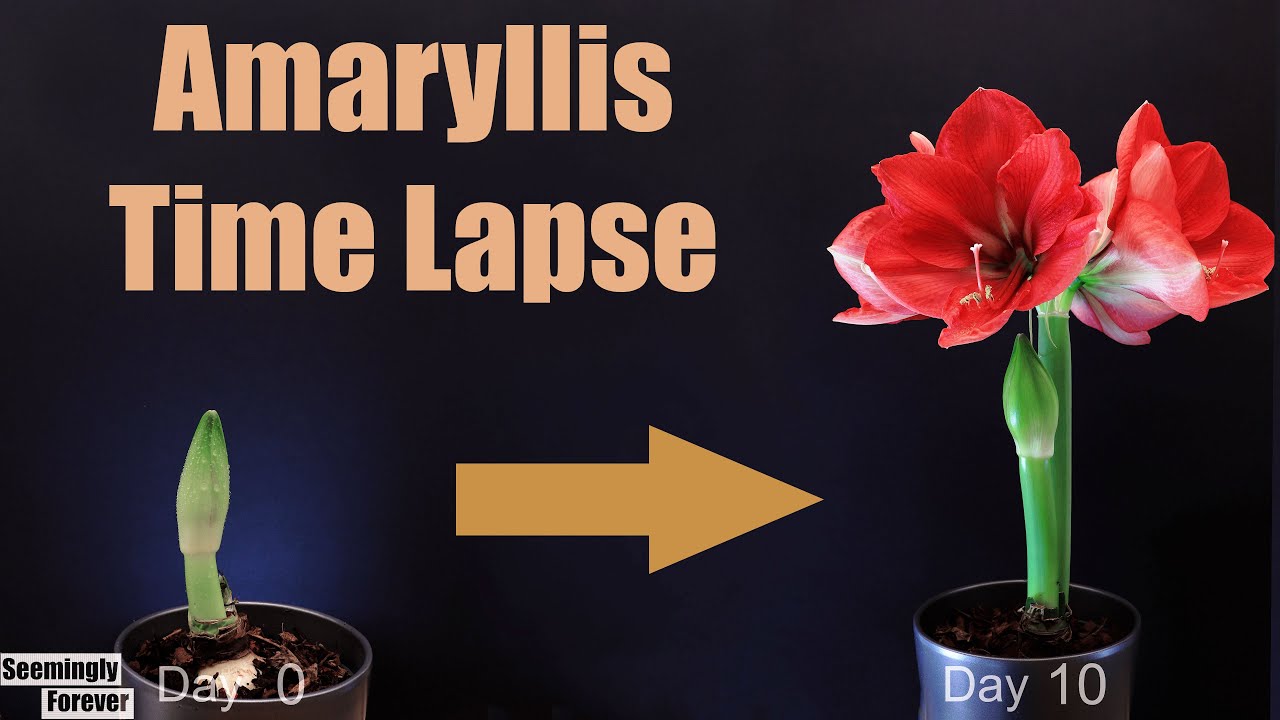This detailed photograph captures the 10-day time-lapse growth of an amaryllis flower, set against a dark navy blue background. At the top, in large peach-pink letters, it reads "Amaryllis Time-Lapse." 

On the left side, the image starts with day zero. Here, we see a small green bud peeking out from the soil in a stylish silver container, about an inch tall. Below it, the text "seemingly forever" appears in a white box, suggesting the anticipation before the bloom. 

An orange-yellow arrow extends from this initial stage, leading the viewer's eye to the right towards the day 10 mark. On this side, the same pot now hosts a lush, blossomed amaryllis. The vibrant red petals stand out against the green stem, now about five inches tall. The fully bloomed amaryllis boasts four striking flowers. 

Front and center, the text "day 10" indicates the transformation. This image beautifully illustrates the significant change of the amaryllis flower over a 10-day period.